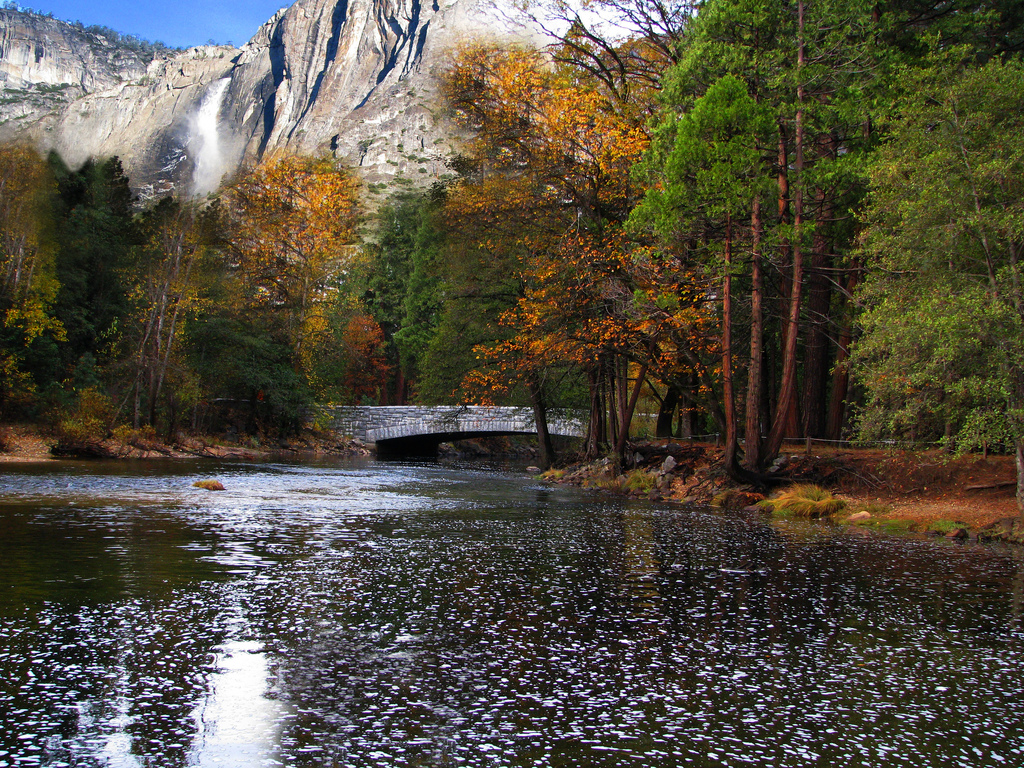The image captures the serene setting of a clear river flanked by a lush array of autumnal trees. The vibrant foliage includes green pines interspersed with trees bearing golden, orange, and red leaves. Prominently, a stone bridge stretches across the river, appearing sturdy enough for vehicular passage. In the distance, the river continues beyond the bridge. To the right, the riverbank is densely populated with trees, while the left bank mirrors this with a similar mix of lush greenery and autumnal hues. Above the river and trees, a gray, mountainous cliff rises majestically, with a white waterfall gracefully cascading down its rugged face, adding to the picturesque landscape. The sky is visible in the top left corner, accentuating the beauty of the outdoor scene.